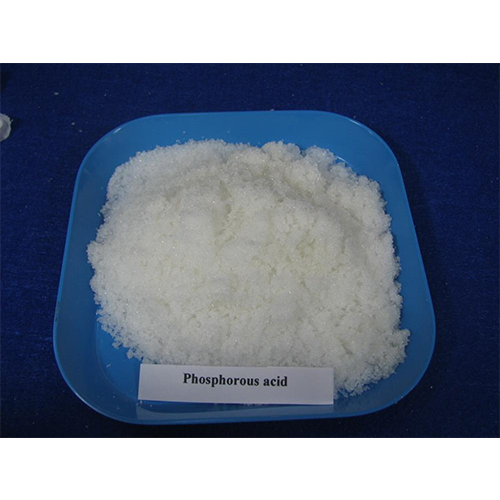The photograph features a square-shaped blue plate with rounded corners, filled to the brim with a large amount of white, crystal-like powder. A white rectangular piece of paper with black printed text reading "Phosphorus Acid" is placed at the bottom of the plate, partially covered by the powder. The blue plate rests on a flat surface that appears to be covered with a blue fabric. The fabric has some specks of white in the top left corner, likely residues of the white substance. Additionally, a white circular object is visible pointing from the left corner of the image. The overall setting suggests a controlled environment, possibly a laboratory, given the presence of the labeled chemical substance.